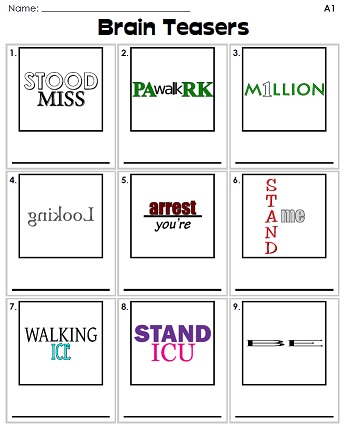The image is a computer illustration resembling a worksheet, likely intended for educational purposes. At the top of the sheet, there's a blank space to write a name, followed by the bold title "Brain Teasers." Below the title, the worksheet is divided into nine distinct boxes, arranged in a 3x3 grid. Each box contains a visual brain teaser puzzle with space at the bottom for the user to write their answer.

Examples of these puzzles include:
- The word "million" where the "i" has been replaced by the number "1," the answer being "one in a million."
- The word "looking" written in reverse, indicating the answer "looking backwards."
- Phrases like "stood" and "miss" creating the puzzle "misunderstood."
- "Paw" aligned with "walk RK," forming the puzzle "pawkward."
- The word "stand" followed by "I see you," suggesting the answer "I see you stand."
- "Walking" with "I see" beneath it, forming "I see you walking."
- The phrase "a rest" on a line, resulting in "a rest."
- "Your" above an apostrophe and "ren," forming "you’re."

Each of these brain teasers encourages the user to think creatively and solve the puzzles by interpreting the visual clues provided.